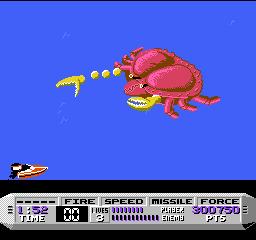This image is a still shot from a retro computer game, characterized by its low resolution and pixelated graphics, reminiscent of old-school game design with a crude and rudimentary aesthetic. The main gameplay area has a solid blue background upon which a cartoonish crab, mostly red with yellow claws and eyes, is prominently displayed. This crab appears to have one claw extended outward, with three spherical yellow objects emanating from it, suggesting either an attack mechanism or some form of interaction.

At the lower part of the screen, there's a distinct status bar featuring a wealth of game-related information. This bar is grey and black with various labeled sections such as "fire," "speed," "missile," and "force," indicating different game metrics or power-ups. A timer is positioned in the lower left corner, reading 1 minute and 32 seconds, marking the urgency of the gameplay under timed conditions. Within the same bar, additional details include the player’s score (300750), the number of lives remaining (three), and a tally of points under different categories such as "player" and "enemy." There is even a small graphic of a motorboat or a similar object near the bottom, which adds to the scene's detail. Overall, this image vividly captures the essence of a classic, nostalgia-evoking gaming experience.